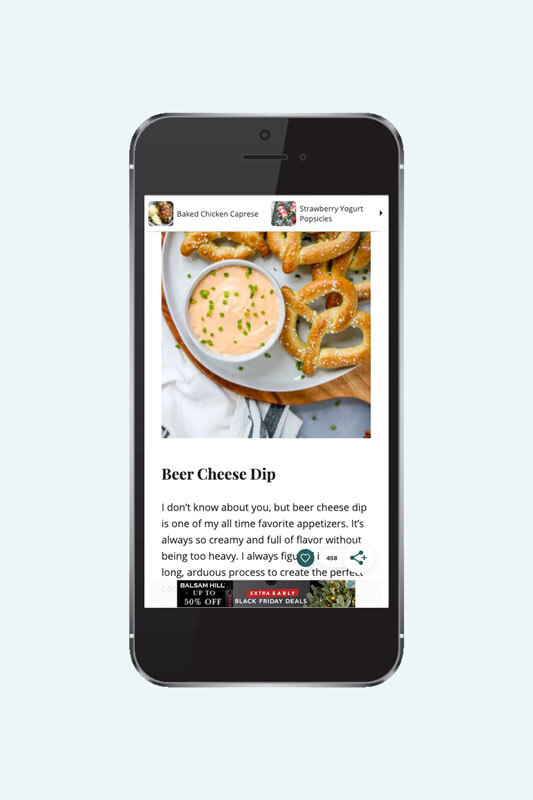In this image, we see an Android cell phone placed centrally on a light teal-gray background. The phone is positioned upright. On the screen, a page displaying a recipe for beer cheese dip is open. The top portion of the screen features a couple of small advertisement images, though their details are indistinct. Dominating the upper half of the screen is a large, square photograph showcasing a blue plate with a bowl of creamy cheese dip on the left, surrounded by several pretzels. Below the image, the text reads "Beer Cheese Dip." The paragraph starts expressing an appreciation for beer cheese dip as a favorite appetizer, lauding its creamy texture and flavorful taste, but the text truncates midway. There are also a few icons, likely for sharing options, and a banner towards the bottom of the screen, containing another advertisement with accompanying images. The phone itself has black sections at the top and bottom, framing the central display screen.